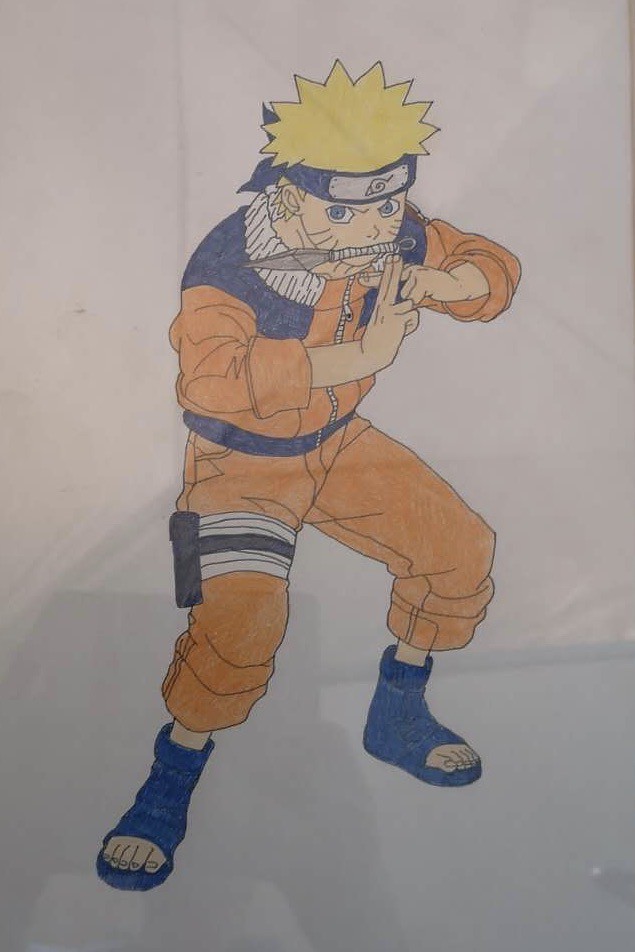The drawing depicts an anime character standing in the center of the image, set against a light blue and pinkish-gray background. The character faces diagonally to the right, exuding a ready-for-action pose with bent knees and feet apart. He has short, spiky blonde hair accentuated by a blue headband wrapped around his head. His striking blue eyes convey intensity, especially as he holds a knife in his teeth, with the blade pointing towards the left side of the picture.

The character’s hands are prominently featured, with his index and middle fingers extended and crossed in a symbolic gesture. He is clad in an orange jumpsuit, paired with blue accents at the chest, collar, and a belt. His footwear consists of blue boots with exposed toes, adding to the ruggedness of his appearance. Notably, a black sheath is secured around his right leg, likely meant for the knife he wields.